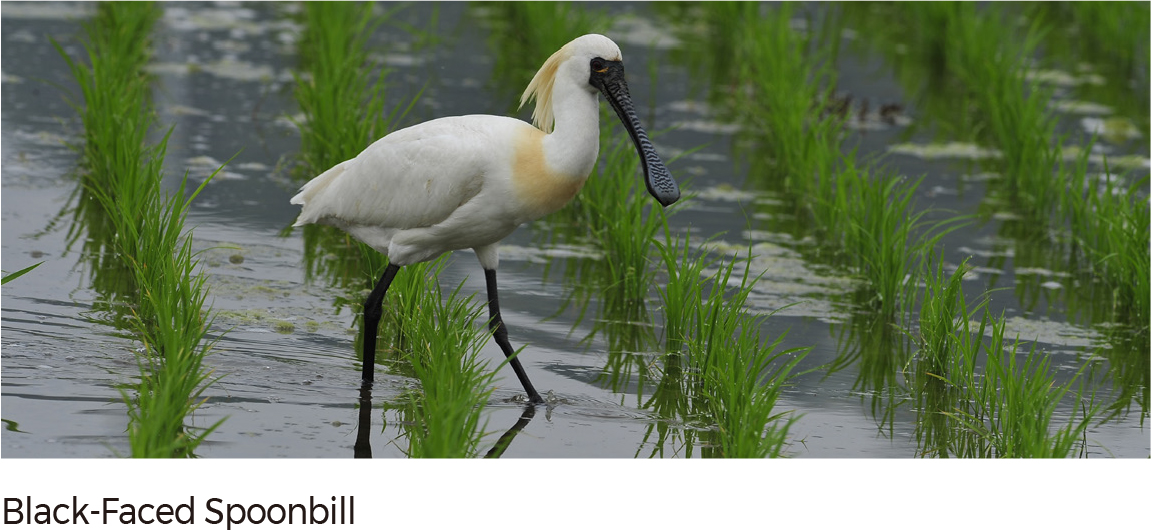This outdoor nature photograph captures a striking black-faced spoonbill bird in a marshy wetland. Shot in a wide-angle, horizontal rectangular orientation, the image features the bird standing centrally, surrounded by a sea of lush green marsh vegetation and water. The bird, shown in profile facing right, boasts a white feathered body with a distinct black face and a long, flat, spoon-like black bill. Thin black legs support its stance in the marsh. Notable yellow feathers stand out at the crest of its head and neck. The detailed close-up leaves no sky or horizon line visible, immersing the viewer in the rich wetland habitat. A black printed caption at the bottom of the photograph reads, "Black-Faced Spoonbill."